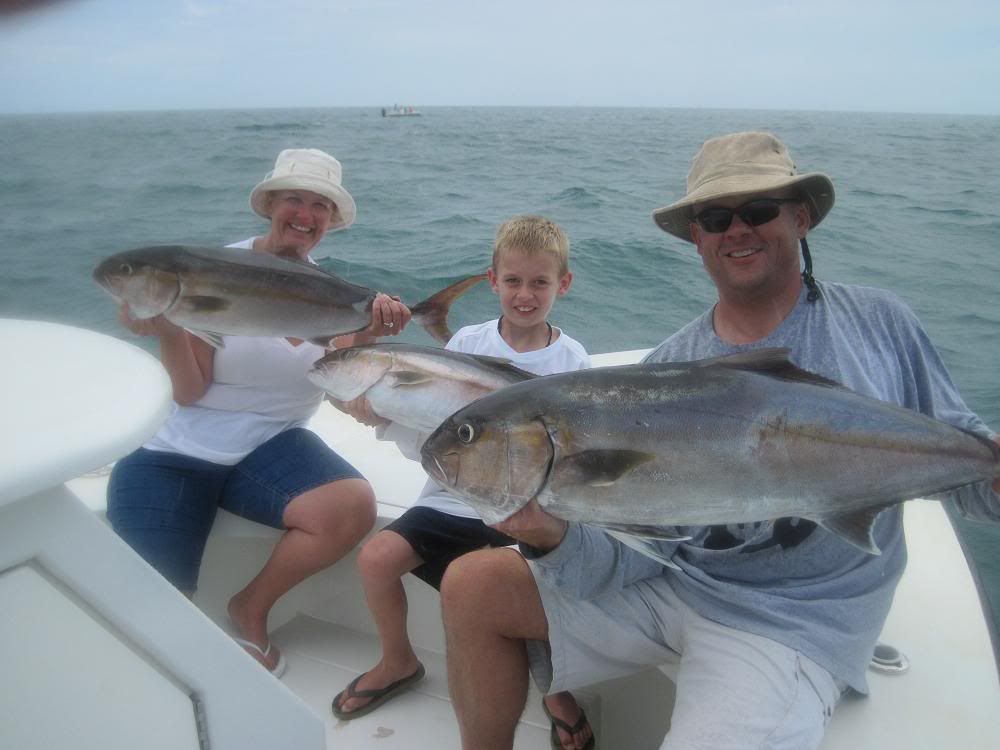In the image, a family of three is joyfully showcasing their fishing success aboard a white boat. The scene captures them in the midst of serene waters, their excitement palpable as they proudly display the large fish they've just caught. The little boy, distinguished by his blonde hair, sports a white t-shirt and olive green flip-flops. He stands beside his mother, who also appears to be blonde, although her hair is partially concealed by a white hat. She is dressed in a white t-shirt, blue jean shorts, and white flip-flops. The father, wearing a gray t-shirt and khaki shorts, completes the trio, his hair hidden under a khaki hat. All three of them are beaming with happiness, their eyes fixed on the camera, while the fish they hold still have their eyes open, adding an eerie yet fascinating touch to the vibrant display of their fishing adventure.